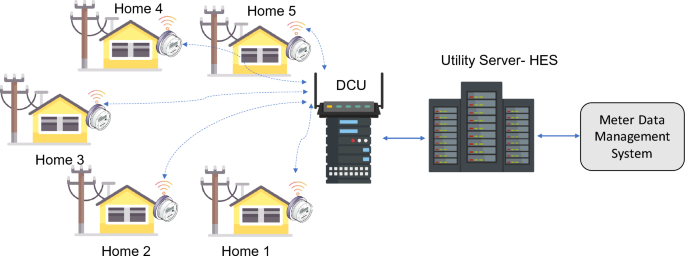The image is a detailed color illustration combined with text, functioning as an informational flowchart on a white backdrop. It visually explains the provision of utility services to homes. Central to the diagram are five identical small yellow homes with brown roofs, side by side in a landscape orientation. Each home is labeled sequentially from Home 1 to Home 5 and has a small utility pole beside it. The flowchart begins on the right with a gray, horizontally oriented rectangle labeled "Meter Data Management System," which features a central panel flanked by smaller ones. From this, a blue arrow points left to a tall, dark gray rectangular illustration labeled "Utility Server-HES." Continuing left, another blue arrow connects to a smaller gray device labeled "DCU," which resembles an electronic box or walkie-talkie with blue stripes. Arrows branch out from the DCU to the five homes, illustrating the path of power distribution from the "Utility Server-HES" to the "DCU" and finally to each home, labeled sequentially from Home 1 to Home 5.